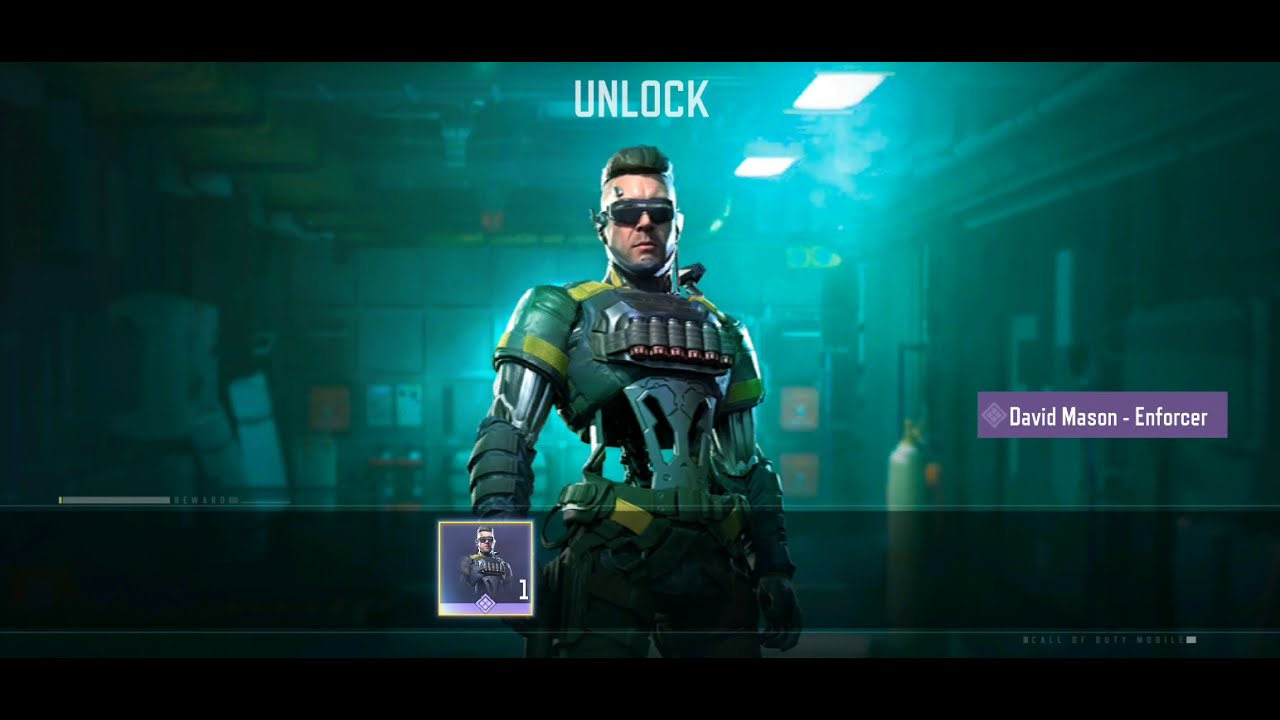The image is a screenshot from a video game featuring a character selection screen. The scene is framed with black bars at the top and bottom. The central figure is a newly unlocked character named David Mason, labeled as "ENFORCER" in a purple rectangle on the right side. The character has a cyberpunk aesthetic, appearing half-man, half-machine with an exposed metallic torso and chest, void of any internal organs or ribcage. He sports dark square sunglasses and a short green mohawk with a shaved side. A chin strap with a mouthpiece or microphone adds to his futuristic look. Significant details include large bullet shells strapped across his chest and enhanced, armored robotic arms. The background resembles a factory with various boxes and shelves. Below the character, a smaller icon of David Mason appears alongside a diamond symbol, and a number 1 is visible in the bottom right corner of the image.